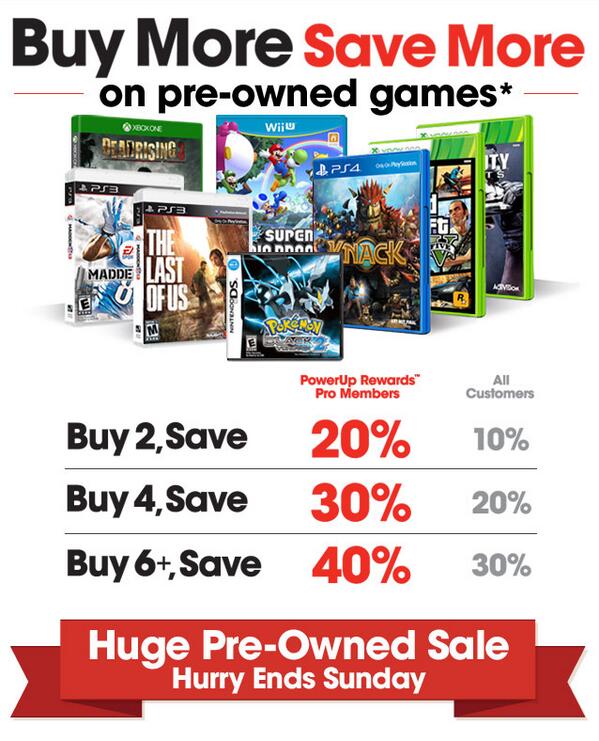**Detailed Advertisement Caption:**

The image features a promotional card for pre-owned video games. The back of the card is entirely white. In the top left corner, bold black text reads, "BUY MORE," while the top right corner displays bold red text, "SAVE MORE." Beneath these headings, black text states, "on pre-owned games*," indicating a footnote exists, though it is not visible in the image.

Prominently displayed are various images of pre-owned game titles, including "Dead Rising," "Madden," "The Last of Us," "Pokemon," "Knack," "Super Mario Brothers," and possibly "Grand Theft Auto." These games are available for a variety of consoles such as Xbox One, PS3, Wii, and PS4.

Below the game images, the offer details are laid out: "Power Up Rewards Pro Members" receive greater discounts, with structures such as "Buy 2 Save 20%," "Buy 4 Save 30%," and "Buy 6+ Save 40%." Contrastly, regular customers who are not part of the membership program save less, with discounts of "10%, 20%, and 30%" for the same quantities.

At the bottom corner of the card, there is a large banner that resembles a red ribbon, featuring indents on both the left and right sides. White text across this ribbon announces, "HUGE PRE-OWNED SALE - HURRY ENDS SUNDAY."

Notably, the phrase "BUY MORE SAVE MORE on pre-owned games" at the top includes an asterisk, implying there is additional information not visible in this image.